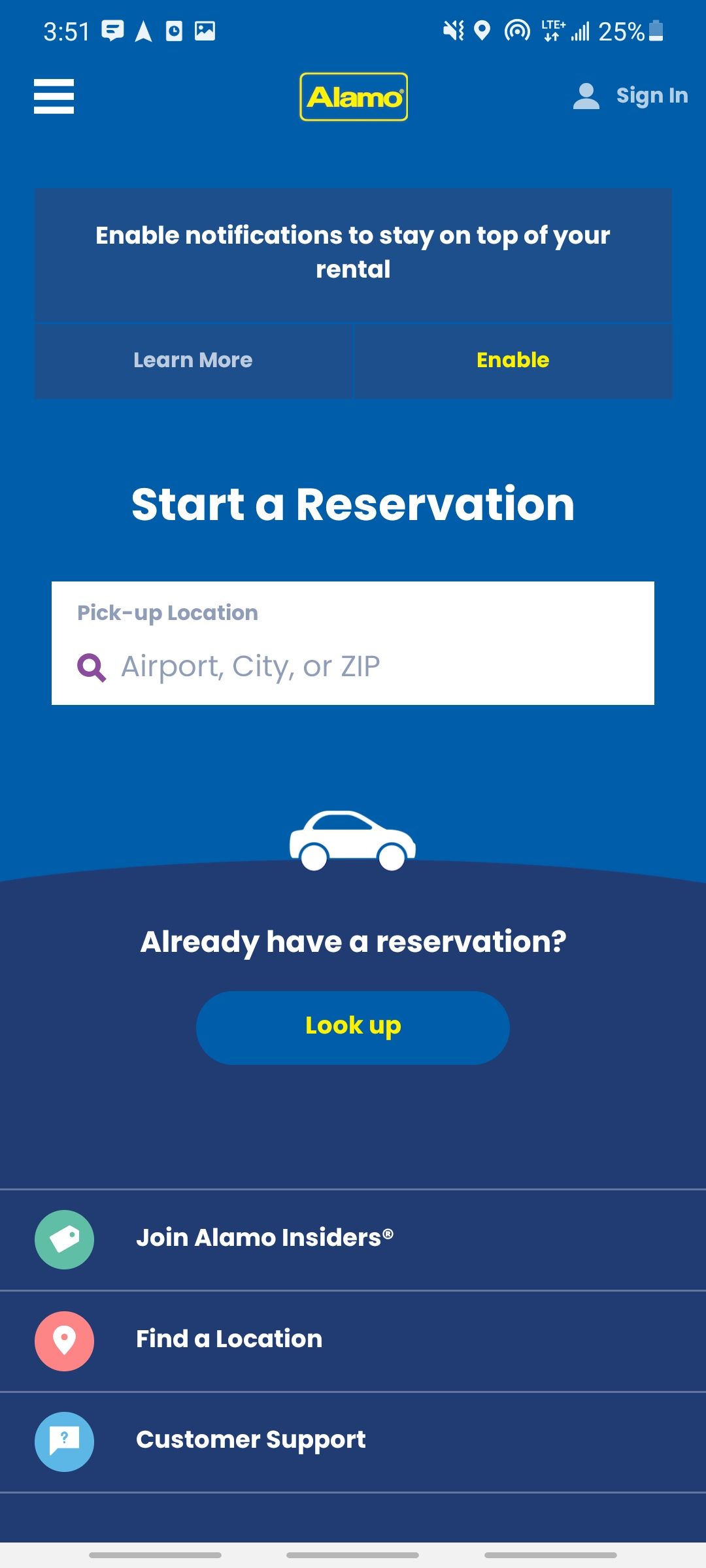A detailed screenshot captures a mobile phone interface against a background gradient that transitions from a lighter blue at the top to a darker blue at the bottom. The phone display indicates a time of 3:51 PM with a battery level critically low at 25%. 

Underneath the status bar, the interface features a prominent hamburger menu icon. Below the menu, the Alamo car rental logo, showcasing their signature blue and yellow colors, appears. The screen offers the option to sign in, and a concise reminder to "enable notifications to stay on top of your rental" is highlighted, with links to either learn more or enable notifications directly beneath it.

Further down, the screen prompts users to start a new reservation by entering their pickup location, including details like the airport, city, or zip code. An animated car icon follows, next to the option "I already have a reservation, look it up," which can be clicked for quick access to existing bookings.

The interface also provides three additional navigational choices stacked vertically at the bottom. The first option, "Join Alamo Insiders," is marked with an identifiable green tag and logo. The second, "Find location," features a coral-colored circle with a pinpoint icon. Finally, "Customer support" is listed for users seeking help.